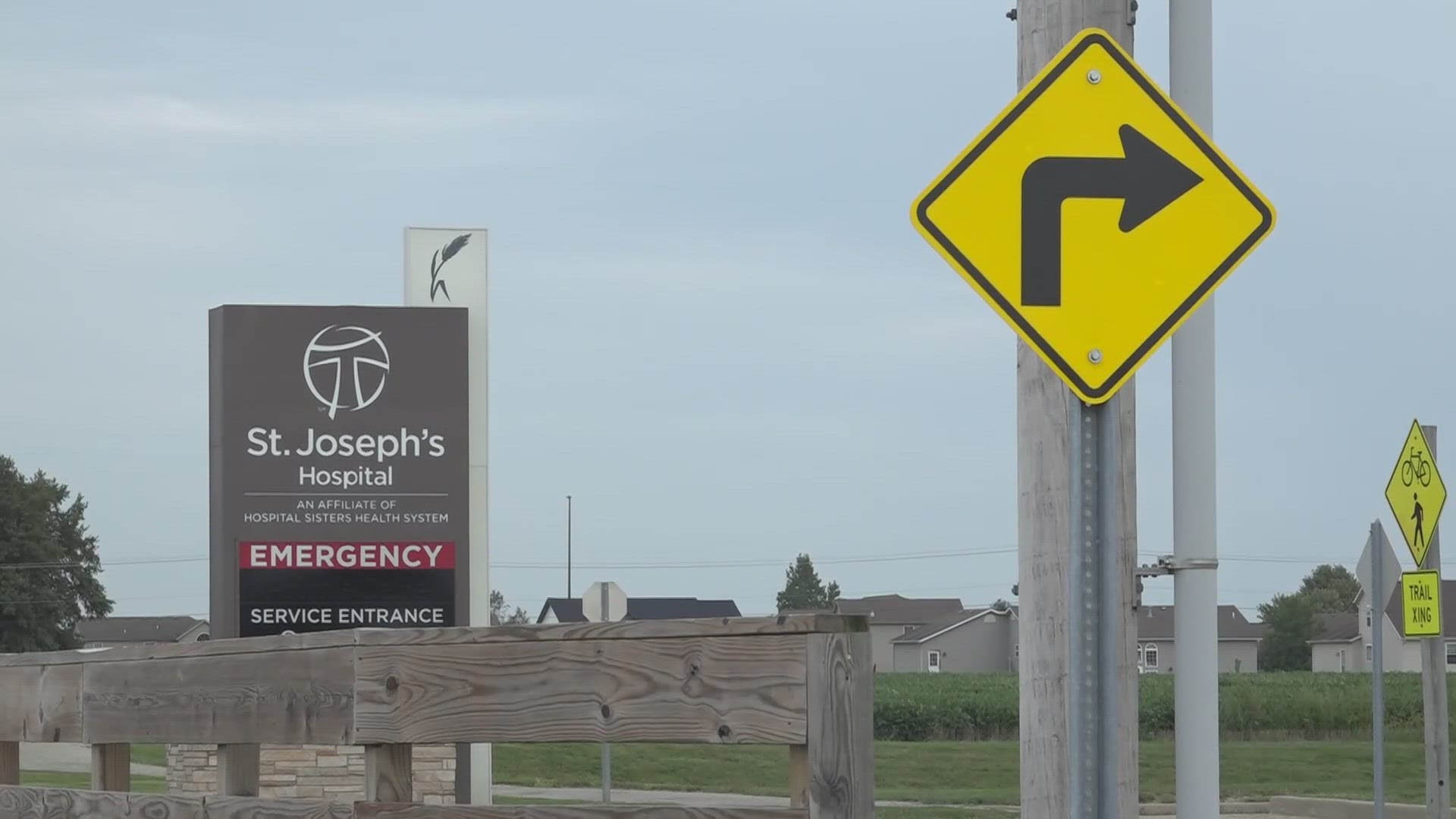The photograph, taken during the day, features a vibrant outdoor scene with a prominent sign for St. Joseph's Hospital. The sky in the background is a mix of light blue and gray hues with thin, wispy clouds. The main sign, which is dark gray with white text, reads "St. Joseph's Hospital, an affiliate of Hospital Sisters Health System," and prominently displays an emergency designation in red. The sign also includes a white emblem that resembles a "T" within a circle.

In the foreground, there is a sturdy wooden fence stretching from the bottom left to the center of the image. Adjacent to this fence are several road signs on poles. To the right of the hospital sign stands a yellow diamond-shaped caution sign with a right-pointing arrow. Further right, nearly at the edge of the frame, is another yellow diamond sign featuring icons of a bicycle over a pedestrian, with a rectangular sign below it that reads "Trail Crossing." Behind these signs, the background shows a neighborhood scene with several houses, adding a sense of community to the hospital's vicinity.